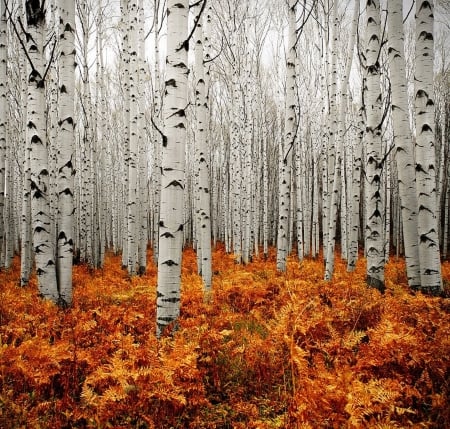The image showcases a dense forest of birch or aspen trees with their distinctive white trunks and black spots, standing tall and slender, extending endlessly into the background. The forest floor is carpeted with vibrant autumn foliage, predominantly orange with hints of red, yellow, and green, creating a striking contrast with the pale tree trunks. The scene is captured in a crisp, neat photograph that emphasizes the stark, leafless trunks and scattered branches. The forest floor appears darker towards the edges, especially on the bottom right and left corners, adding depth to the composition. A glimpse of white sky is visible in the background, though it is mostly obscured by the numerous tree trunks that lead the viewer's eye deep into the forest. The overall effect is a stunning interplay of autumn hues and the monochromatic elegance of the tree trunks.